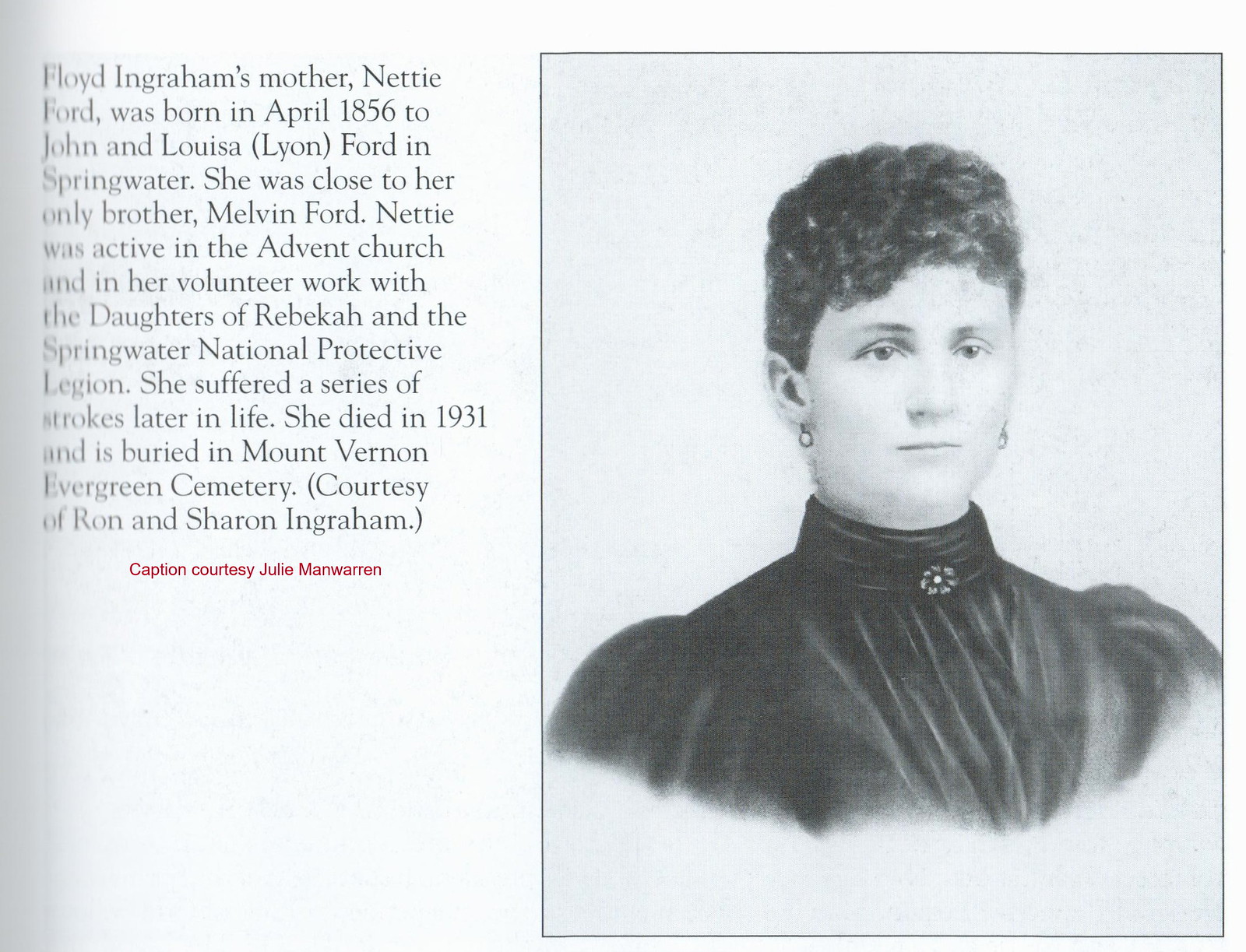This image appears to be a black and white scan of a book page printed on white or light-blue cardstock. Featured prominently on the right side is a photograph or a very detailed sketch of a woman from the late 1800s or early 1900s. The woman, identified as Floyd Ingram's mother, Nettie Ford, has short curly hair and is adorned with small earrings. She is dressed in a black turtleneck dress with a small brooch or flower on the collar and stands against a white background. The image appears to fade out towards the bottom and left. 

The text accompanying the image, stated twice in red print, offers biographical details about Nettie Ford. It reads: "Floyd Ingram's mother, Nettie Ford, was born in April 1856 to John and Louisa Lennon Ford in Springwater. She was close to her only brother, Melvin Ford. Nettie was active in the Advent Church and in her volunteer work with the Daughters of Rebecca and the Springwater National Protective Legion. She suffered a series of strokes later in life and died in 1931. Nettie is buried in Mount Vernon Evergreen Cemetery." The caption is credited to Julie Mann-Warren, with the courtesy of Ron and Sharon Ingram.